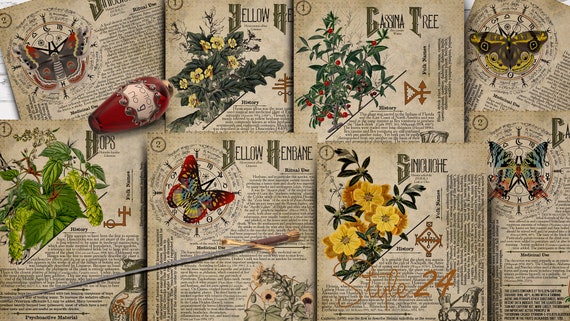This image depicts a meticulously arranged collage of old book or magazine pages, each featuring botanical and entomological illustrations, primarily of flowers, plants, and butterflies. The pages, giving off a sepia or golden hue, evoke an antique style reminiscent of 19th or early 20th-century print. The spread contains about six or seven different pages, positioned in two rows, with the top row extending from the top left to the top right and a second row beneath. Among the plants and butterflies, specific text captions can be seen, including phrases like "yellow urn brain," "gossam tree," and "yellow henbane." The illustrations include yellow flowers with green leaves, cherry-like blossoms, and detailed butterfly diagrams. There are instances of cursive and ornate old-fashioned text headings, enhancing the vintage aesthetic. Additionally, the image includes a small, old knife and a tipped bottle, lending a further sense of antiquity and curiosity to the scene. The vivid color palette spans greens, dark greens, yellows, reds, beiges, tans, grays, blacks, and whites.